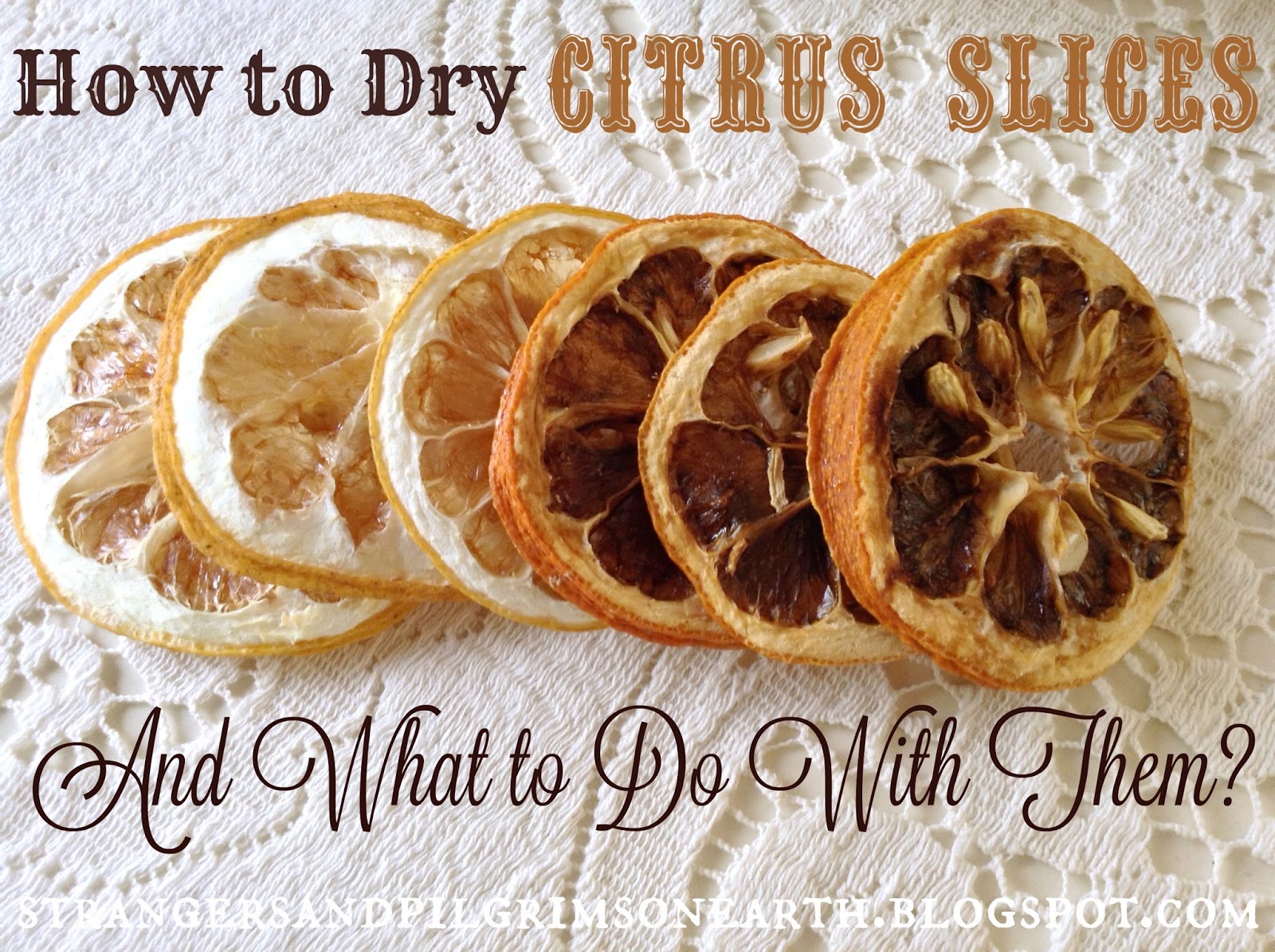This rectangular photograph serves as an instructional visual guide on how to dry citrus slices. The image is on a white doily backdrop that appears slightly off-white. At the top, it features the title "How to Dry Citrus Slices" with "how to dry" in a dark brown font and "citrus slices" in a larger, dark orange, all-caps font. Below this heading, a series of six orange slices span from left to right, progressively appearing drier. The slices on the left are nearly fresh with a vibrant, bright orange peel and a mostly white and orange interior. Moving rightward, the slices transform in dryness, with the last three taking on a dark amber hue inside and a much darker orange peel. Below these images, in elegant black cursive, is the caption "and what to do with them." At the very bottom in white, all-caps font is the web address "strangersandpilgrimsonearth.blogs.com," which contrasts against the off-white background. The attention to detail and gradual change in the appearance of the citrus slices vividly illustrate the drying process.